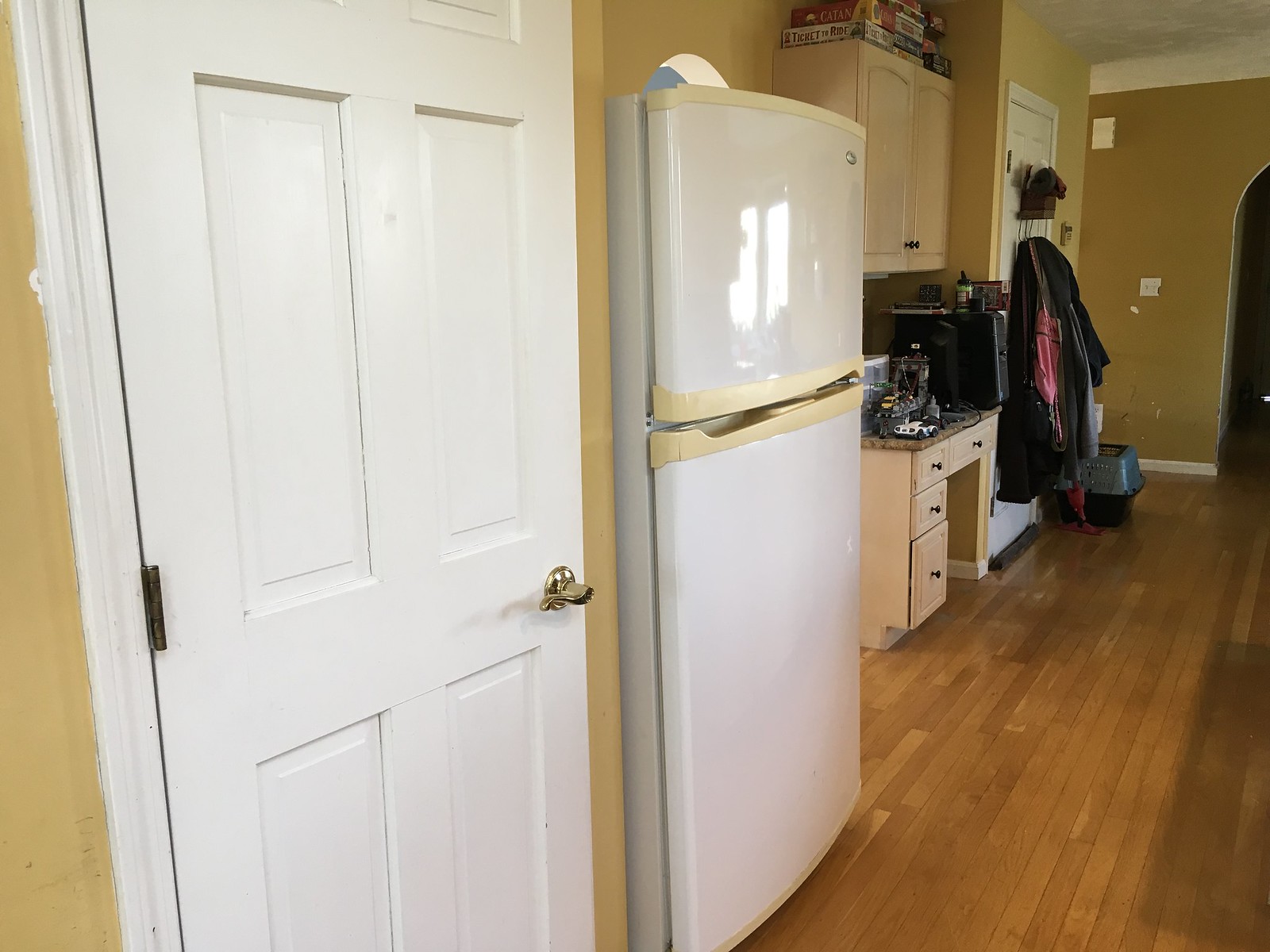This photograph captures the interior of a somewhat rundown kitchen. The scene is dominated by medium-colored wood plank floors and walls poorly painted in a gold hue, framed by white trim. Closest to the viewer on the left is a white panel door with a gold handle. Adjacent to the door is a two-door refrigerator, with a yellowed strip of plastic between the top freezer and bottom fridge compartments. 

Moving further into the room, there is a built-in desk with clutter on a counter beneath it, along with cabinetry above the desk that is topped with stacks of board games, including titles like Ticket to Ride and Catan. To the right of the desk, another door is visible with several coats hanging from hooks. 

In the far end of the kitchen, a darker mustard or brown wall features crown molding and a white light switch. There is also a pet carrier and a floor sweeper nearby, adding to the room's cluttered feel. The photograph shows a white ceiling, and to the far right in the back, an archway marks the entrance to another room.